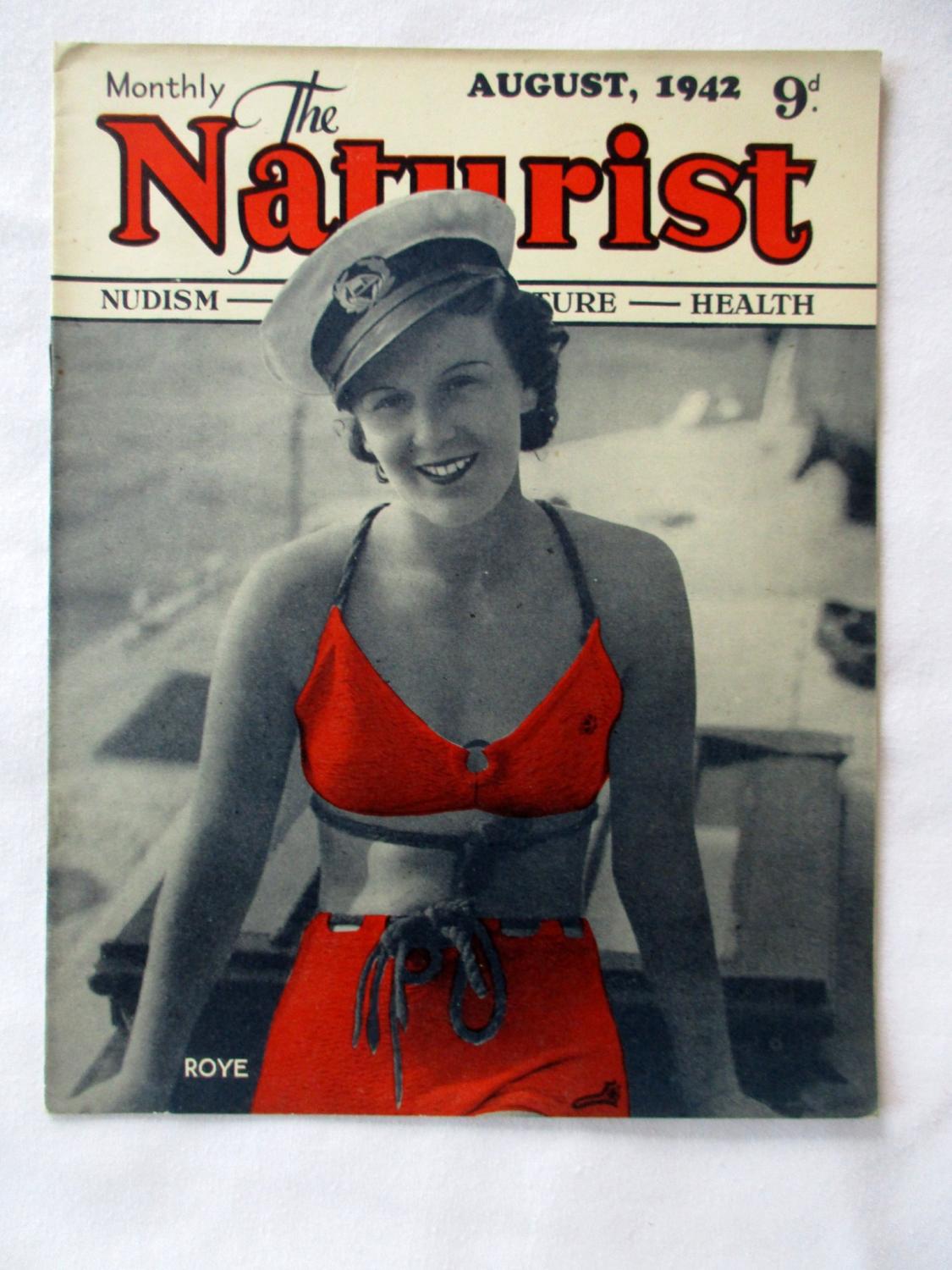The image depicts a vintage magazine cover, aged and in black and white, with deliberate digital alterations adding vibrant red accents, creating a striking pop art effect. At the top, the text reads "The Naturist" or possibly "Naturist." To the left, beneath this title, the word "Nudism" appears, while "Health" is inscribed on the right. Central to the cover is a woman, seemingly depicted in the nude, but she has been digitally dressed in a bright red bikini that starkly contrasts with the original monochromatic scheme, lending a modern, surreal twist to the vintage aesthetic. In the upper right corner, the date "August 1942" is visible, along with the price listed as "9 cents." The lower corners of the cover feature additional details: the lower left corner bears the name "Roy," likely attributing credit to the photographer. This intricate blend of past and present offers a fascinating glimpse into both historical publication design and contemporary artistic reinterpretation.